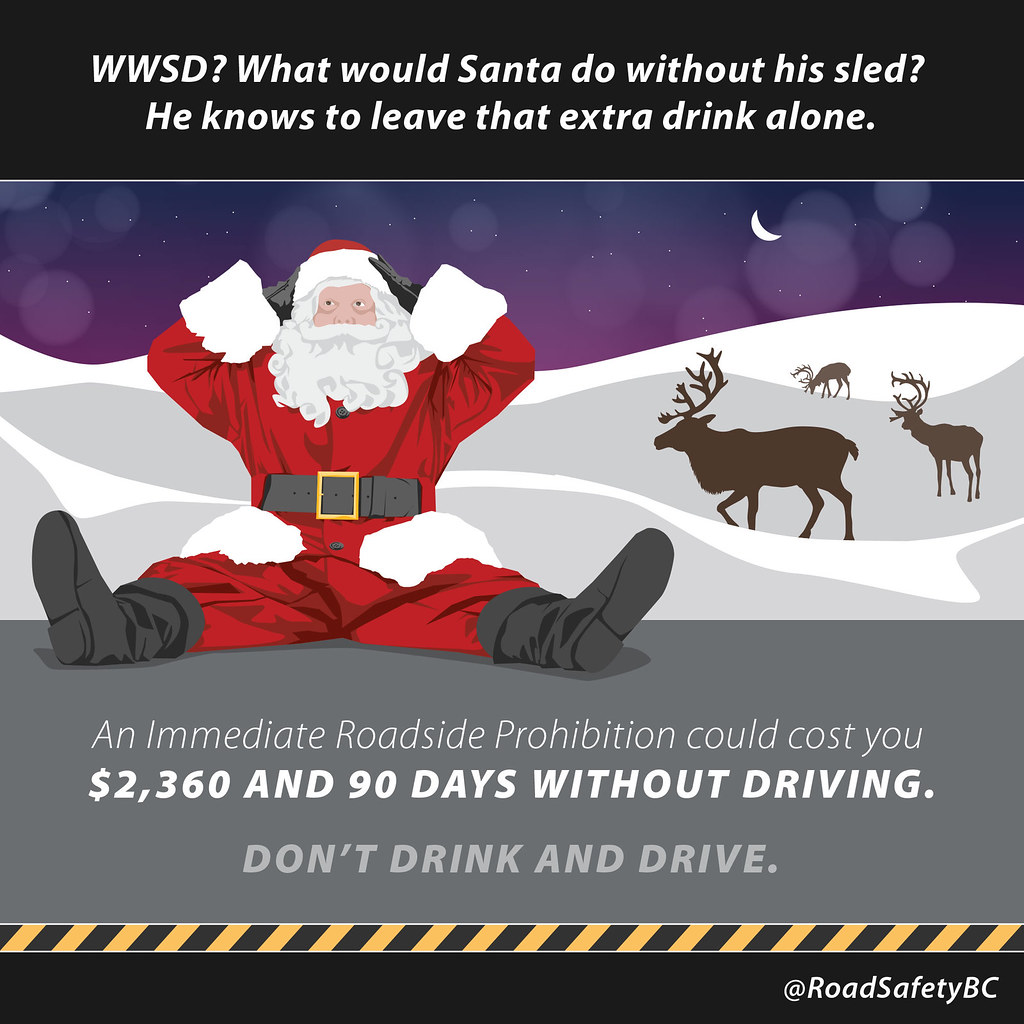This cartoonish advertisement is a cautionary message about not drinking and driving, featuring Santa Claus against a purple, pink, and blue night sky adorned with a crescent moon and stars. The image is framed with a thick black header and footer. The header, in white text, reads: "WWSD? What would Santa do without his sled? He knows to leave that extra drink alone." Santa, dressed in his iconic red suit, is depicted sitting on a pavement with his hands on his head and legs extended in front of him, surrounded by snowbanks. Behind Santa, three brown reindeer graze in the snow. Notably, Santa exclaims, "What have I done? I've lost my sled. There'll be no Christmas now because I was drinking and delivering presents in my sleigh."

In white text on the road beneath Santa, the warning states: "An immediate roadside prohibition could cost you $2,360 and 90 days without driving." Below that, in gray print, the message "Don't drink and drive" is emphasized. At the very bottom of the image, a black and yellow caution banner runs across, with the advertising organization's name, "RoadSafetyBC," marked in white text in the lower right corner. This poignant and vivid portrayal aims to remind viewers of the serious consequences of drinking and driving, potentially ruining even Santa's Christmas.